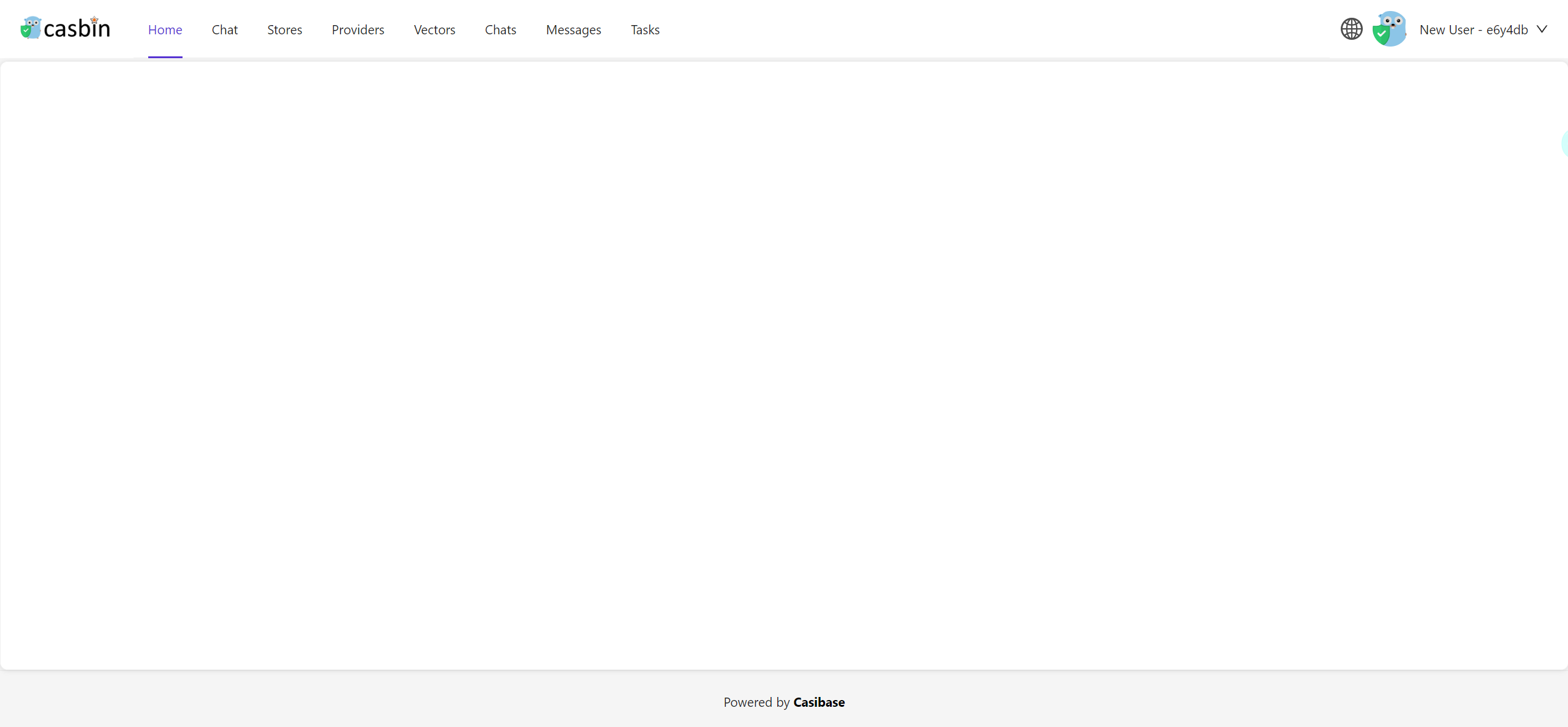This image is a detailed screenshot of a computer page interface. In the upper left corner, the text "Caspian" is displayed in black, accompanied by a small blue trash can icon to its left. The top navigation bar includes several tabs: Home, Chat, Stores, Providers, Vectors, Chats, Messages, and Tasks. The "Home" tab is highlighted in blue and underlined with a blue line, indicating it is the current active page.

On the upper right side, there is a circular icon with what appears to be small squares inside it, next to a blue owl icon with a green checkmark adjacent to it. The text "New User E6Y BDB" is displayed beside a dropdown arrow, suggesting user account options.

The central portion of the screen is dominated by a large, empty white rectangular area, devoid of any images or people. This suggests that the main content area is currently blank or waiting to load.

Finally, at the very bottom of the page, there is a gray border. Centrally placed within this border is the text "Powered by CassieBase," indicating the technical foundation of the interface.